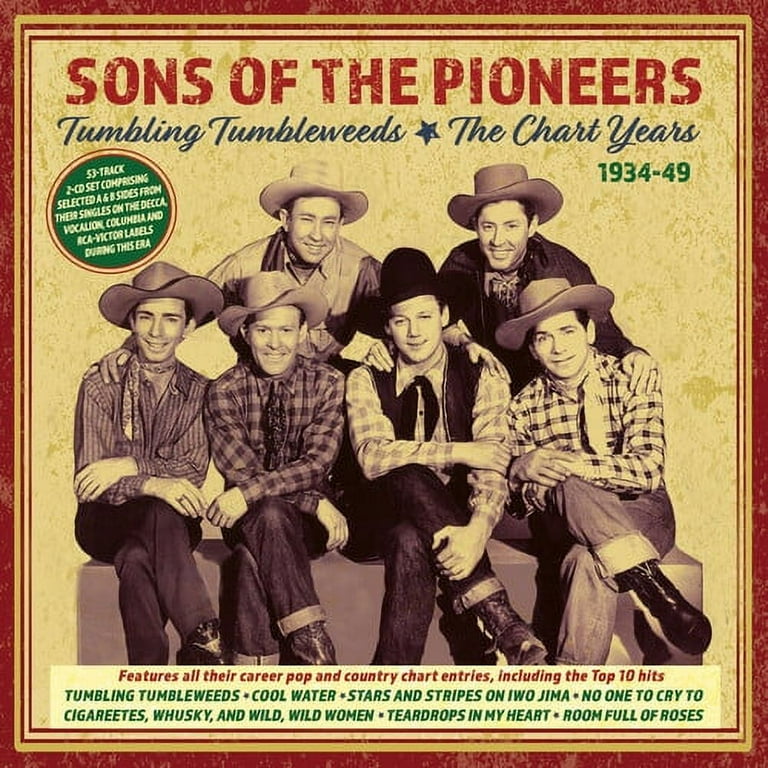This vintage album cover for "Sons of the Pioneers: Tumbling Tumbleweeds - The Chart Years 1934-1949" strikes a nostalgic chord with its distinctive design and detailed artistry. The cover features a dull yellow background encased within multiple borders, alternating between red and yellow, culminating in a vibrant outermost red border. At the top, the title "Sons of the Pioneers" is prominently displayed in red letters, followed by "Tumbling Tumbleweeds" in blue. Below, a green circle highlights the years "1934-1949" and indicates that the album is a "53 track 2 CD set comprising selected A and B sides from their singles on the Decca, Vocalion, Columbia, and RCA Victor labels during this era." 

At the heart of the cover, the six members of the Sons of the Pioneers are depicted, embodying the quintessential cowboy look. The two men in the back and four men in the front are all adorned in cowboy hats, flannel long-sleeve, checkered or button-up shirts, jeans, and cowboy boots. Some of them wear different types of bandanas tied around their necks, adding to their rugged charm. Their attire complements the vintage Western theme, enhancing the nostalgic feel of this iconic album. Below the image of the group, a list of their classic songs is featured, including "Tumbling Tumbleweeds," "Cool Water," "Stars and Stripes," "On to Gemma," "No One Cried Two Cigarettes," "Rusky and Wild," "Wild Woman," "Teardrops in My Heart," and "Room Full of Roses."